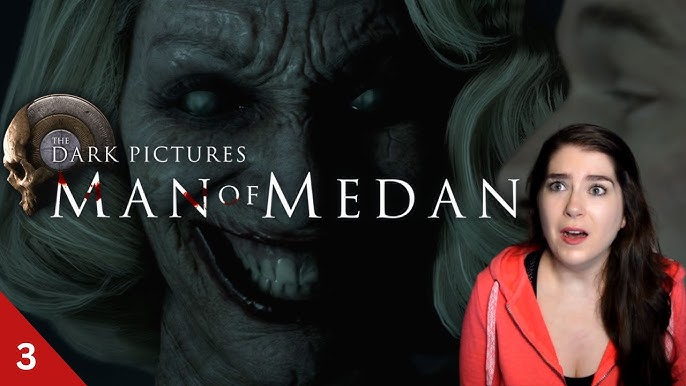The image is a full-color, rectangular movie poster titled "The Dark Pictures: Man of Medan." This title appears in large white text, centered in the middle of the image with a gray circle enclosing a sideways skull. Dominating the lower right corner is a white woman with long, dark hair parted to her left. She has a shocked expression with wide-open eyes and mouth, wearing a red-orange hoodie over a low-cut black crop top, revealing some cleavage. In the lower left corner, a small red triangle features a white numeral three. The background faintly shows a menacing statue or monster with a wrinkled face, big teeth, and a sinister smile, having white eyes with no pupils and short, curled blonde hair.